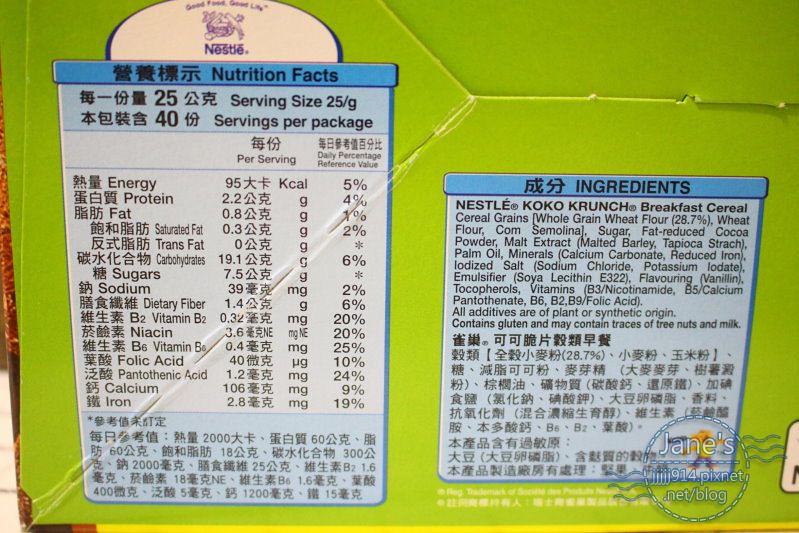This rectangular image showcases a close-up photograph of a cardboard package, likely viewed from the side or bottom. The packaging features a distinctive lime green color with blue labels. Diagonal folds run from the lower left towards the upper right, adding to the texture of the cardboard. Prominently displayed on the label are Asian characters alongside English text. Nestle's logo, printed in blue, appears above the nutrition facts which specify a serving size of 25g and a total of 40 servings per package. Detailed nutritional information lists energy, protein, and fat content. 

On the right side of the label, against a blue background, the ingredients are clearly visible: Nestle Cocoa Crunch Breakfast Cereal, comprising cereal grains like whole grain wheat flour, wheat flour, corn semolina, sugar, fat-reduced cocoa powder, and malt extract. In the lower right corner, a round watermark in white text reads "Jane's jjjjjj914.pixnet.net/blog," adding a unique touch to the packaging.